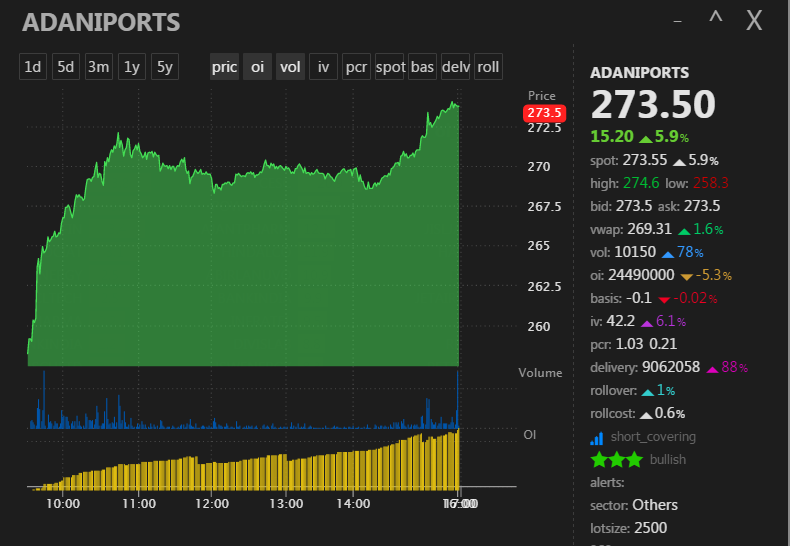The image displays a financial tracking window against a black background. In the upper left corner, there is a closed box, an upward caret, and an underscore symbol, likely representing options to close, maximize, or minimize the window. On the far left at the top, the title "ADANIPORTS" is prominently displayed, indicating that the data pertains to Adani Ports.

The main content of the window features a detailed line graph tracking the investment performance of Adani Ports. The graph showcases a jagged green line, representing price fluctuations, with a lighter green area filled in beneath the curve for visual clarity. The graph is supplemented by various time frame controls at the top, allowing for adjustments to display data over one day (1D), five days (5D), three months (3M), one year (1Y), or five years. Additionally, users can select different types of graph data, including price, open interest (OI), and volume.

Below the primary line graph, a volume graph is depicted with blue vertical lines indicating the number of shares traded each day. Alongside this, yellow bars represent open interest (OI), although the specific meaning of open interest is not clarified. 

To the right of the graphs, current statistical data is displayed: the current price of Adani Ports is 273.50, reflecting a rise of 15.20, or 5.9%. The spot price is listed as 273.55, providing instant insight into stock performance. The entire layout is designed to give a comprehensive and visually appealing overview of the Adani Ports stock data.